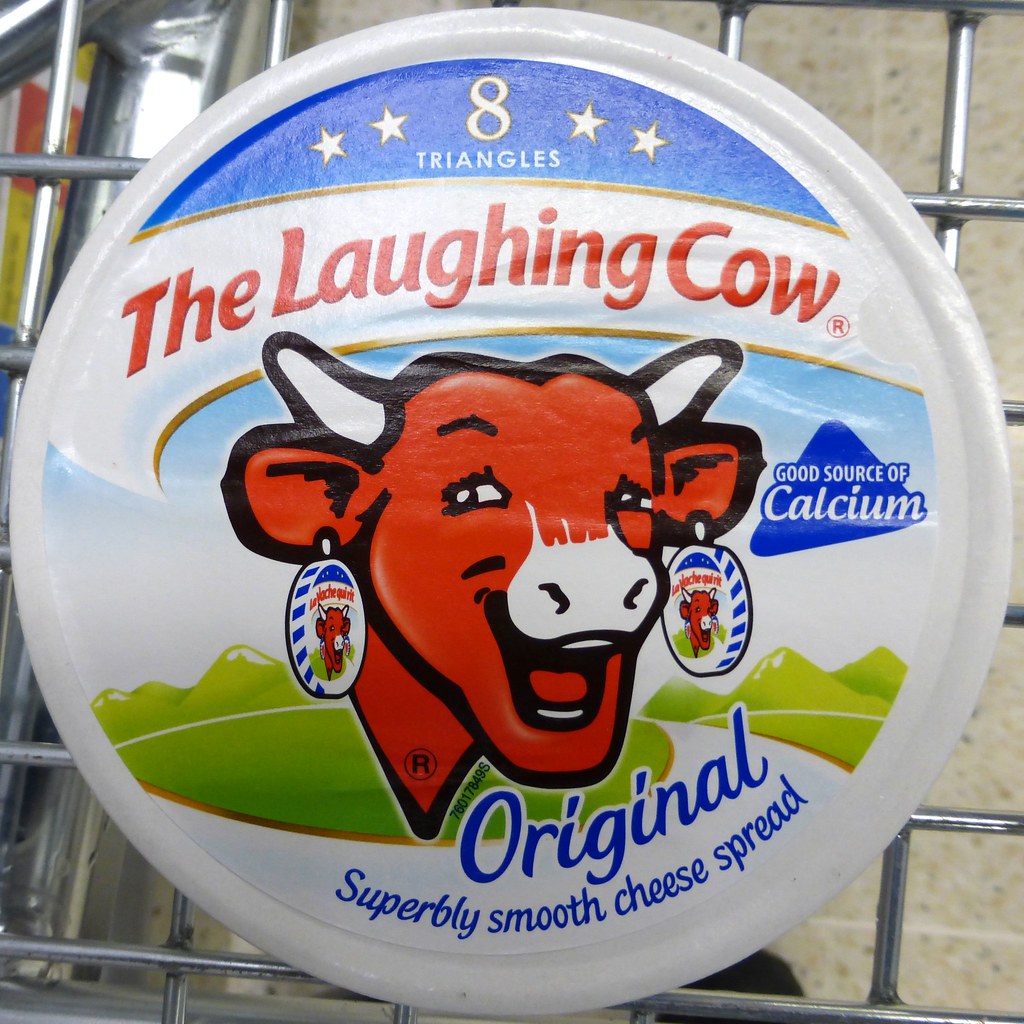The photograph captures a top-down view of a circular cheese spread container placed in a metal shopping cart. The container features a white cap with an intricate paper label. Dominating the label is an illustration of a laughing red cow's head, complete with distinctive white ears and a white nose, and adorned with matching earrings that reflect the product branding. Across the top of the label, in bold red font within a white banner, is the name "The Laughing Cow." Surrounding the cow's image are green cartoon hills with a white road leading forward. Below the cow, in blue text, it states "Original Superbly Smooth Cheese Spread." A blue triangular section on the right side of the cap highlights that the product is a good source of calcium. Two golden stars flanking the number 'H' also feature prominently on the cap, adding to its decorative details.